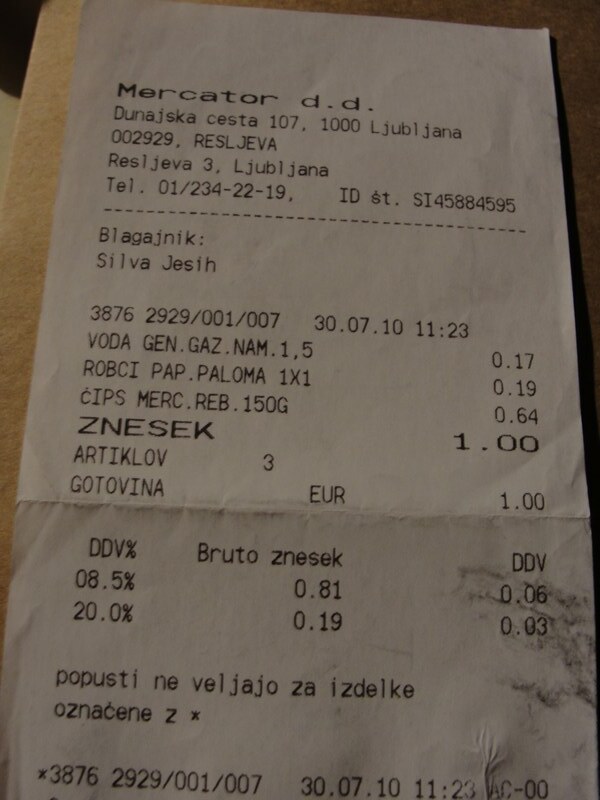This close-up photograph captures a wrinkled white receipt, prominently placed on a beige or tan wooden tabletop, possibly in Eastern Europe. The receipt, with a noticeable crease in the middle, is from a place called Mercator DD. Written at the top in bold black text is "Mercator DD" followed by an address "Dunajska Cesta 107" in an unfamiliar language hinting at its foreign origin. The city name, "Ljubljana," is spelled out in capital letters. The receipt displays an itemized list and a total transaction amount of one euro, accompanied by a tipping suggestion at the bottom. Additionally, there is some smudged grayish-black text in the bottom right-hand corner.